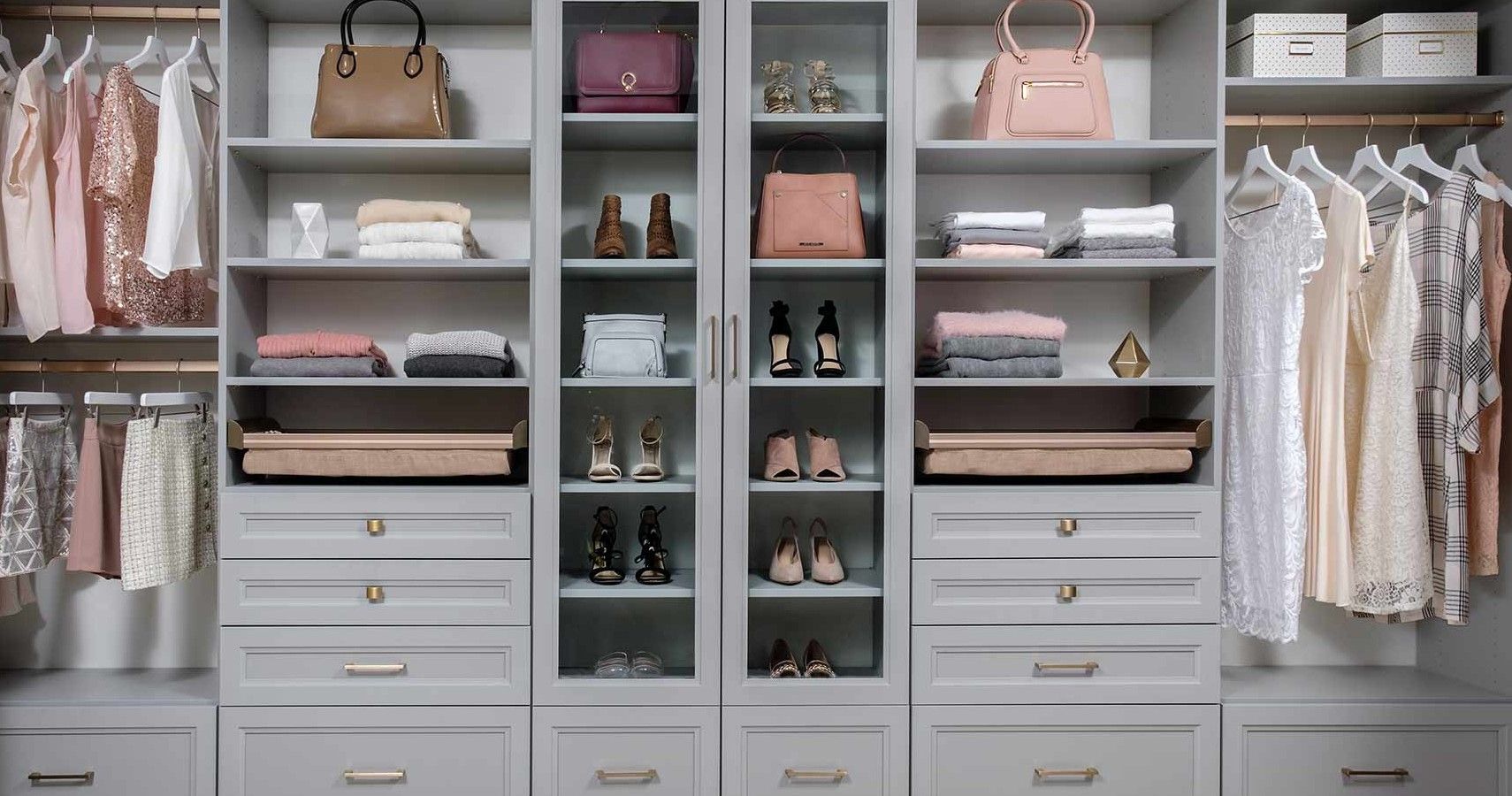This photo captures a well-organized, luxurious female closet featuring an array of wooden cabinetry in shades of gray and white, accented with gold handles. On the left side, blouses and shorts hang neatly on white hangers above drawers, which add to the streamlined look. There are multiple shelves displaying items in meticulous order: a tan luxury purse in a vertical position, various folded shirts in shades of red, blue, plaid, and gray, and a selection of towels in gray, pink, white, and cream. Near the bottom, individual compartments house pairs of shoes, while the upper section showcases more shirts and skirts. The overall aesthetic is elegant, spacious, and adheres to a predominantly neutral color scheme with subtle pops of pink and red.